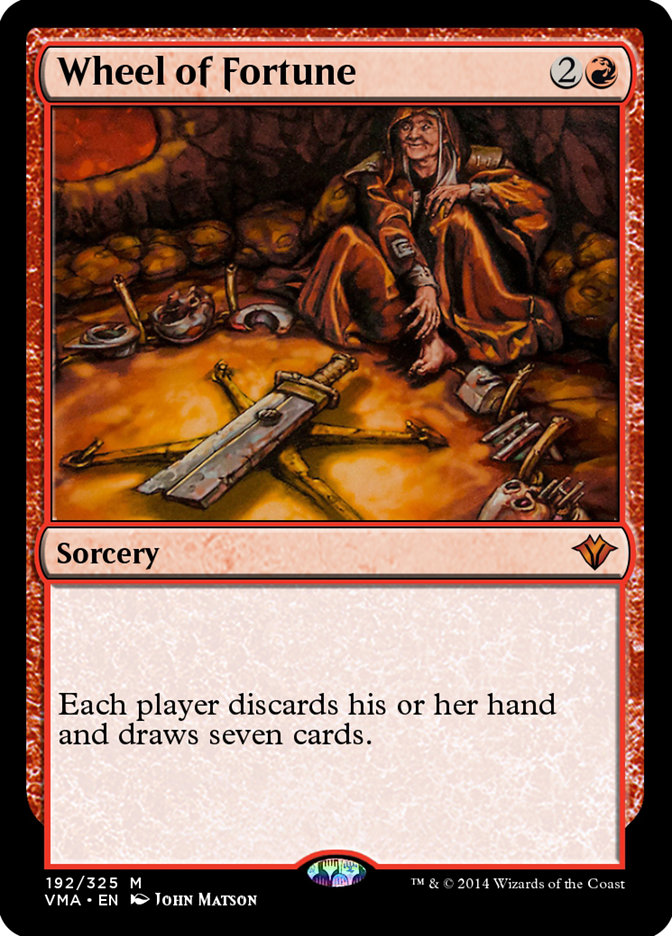The image displays a card likely used in a game, bordered by a black outline within a red frame. At the top, the card features a beige bar with "Wheel of Fortune" in black letters. Below that is a depiction of a figure seated in a cave-like environment. The central character, illustrated with a cartoonish yet detailed style, wears a long orange-brown robe and a hooded cape, and has long white hair. The figure is surrounded by various items, including a broken sword forming an X, bones in bowls, and scattered weapons on an orange floor, with brown walls behind. In the middle section, there's a large circle bearing the number 2 and another with a black image, both outlined in thin red lines. At the bottom of the image, in another beige bar, it reads "Sorcery" followed by "Each player discards his or her hand and draws seven cards." The bottom black border of the card includes the text "192/325 M VMA, TM & © 2014 Wizards of the Coast."